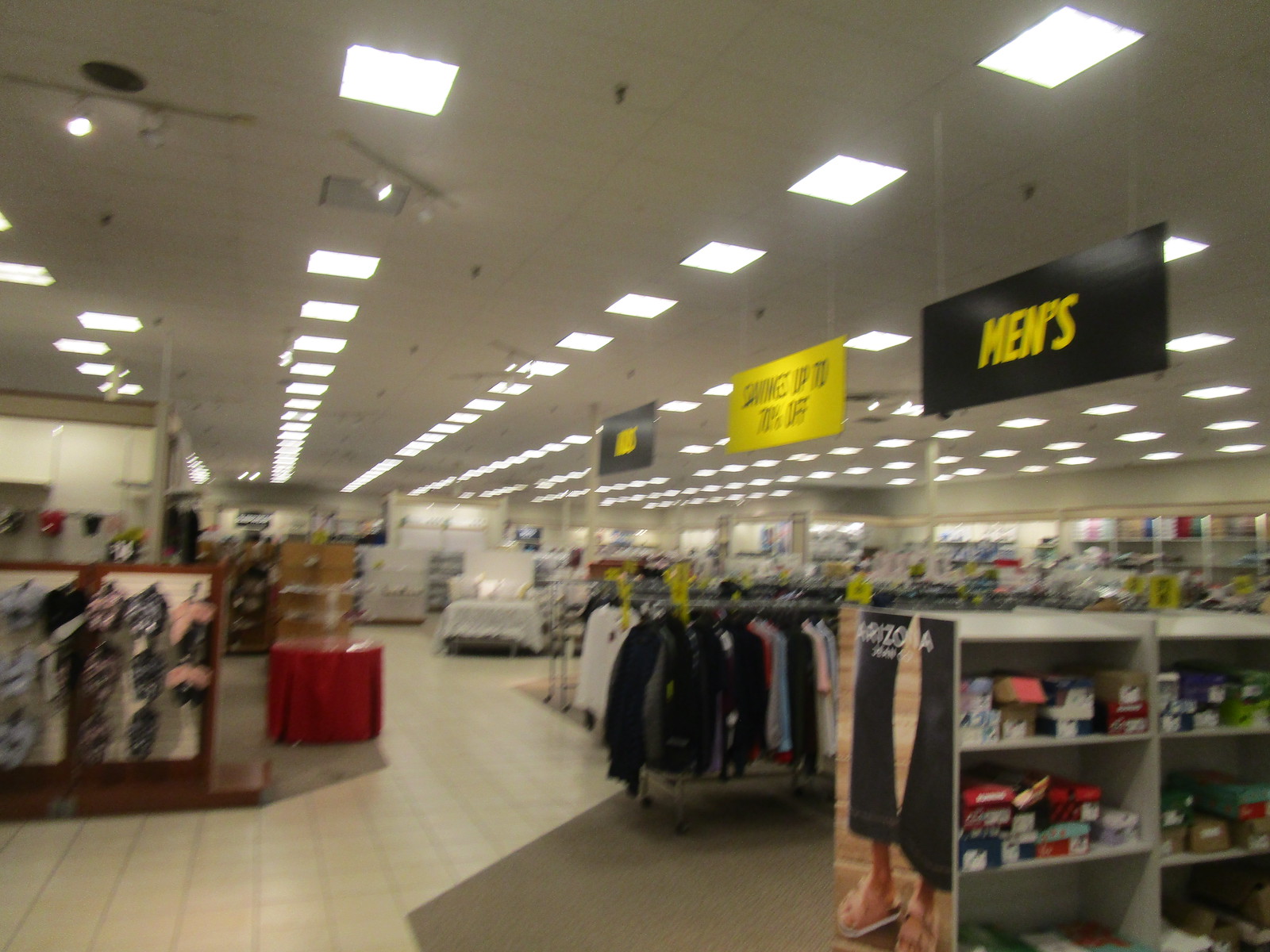This slightly blurry photograph captures the interior of a large department store with very high white, foam-paneled ceilings and long halogen lights set behind plastic tiles that extend from the front to the back of the image. The focal point is a gray display case in the foreground, filled chaotically with shoe boxes of various colors including red, blue, and white. Nearby, a black sign with a yellow "Men's" tag hangs prominently from the ceiling.

At the end of the shoe display, there is an Arizona Jeans Co. poster showing a woman’s legs clad in blue jeans and strapped sandals. Behind this poster, rows of clothing racks hold long sleeve shirts, jackets, and other apparel, with some shelves showing neatly folded shirts. Adding to the store's bustling atmosphere, several black and yellow rectangular signs hang from the ceiling along the right side, one notably mentioning “Savings up to 70% off.”

The store floor transitions from light beige tiles to areas of beige carpet where merchandise is displayed. Along the left side of the image, flip flop sandals hang on a display, while more racks and shelves suggest further assortments of goods, possibly including bedwear. The angular walkway defined by the contrasting flooring leads further into the store, amplifying the expanse and variety of the shopping space.